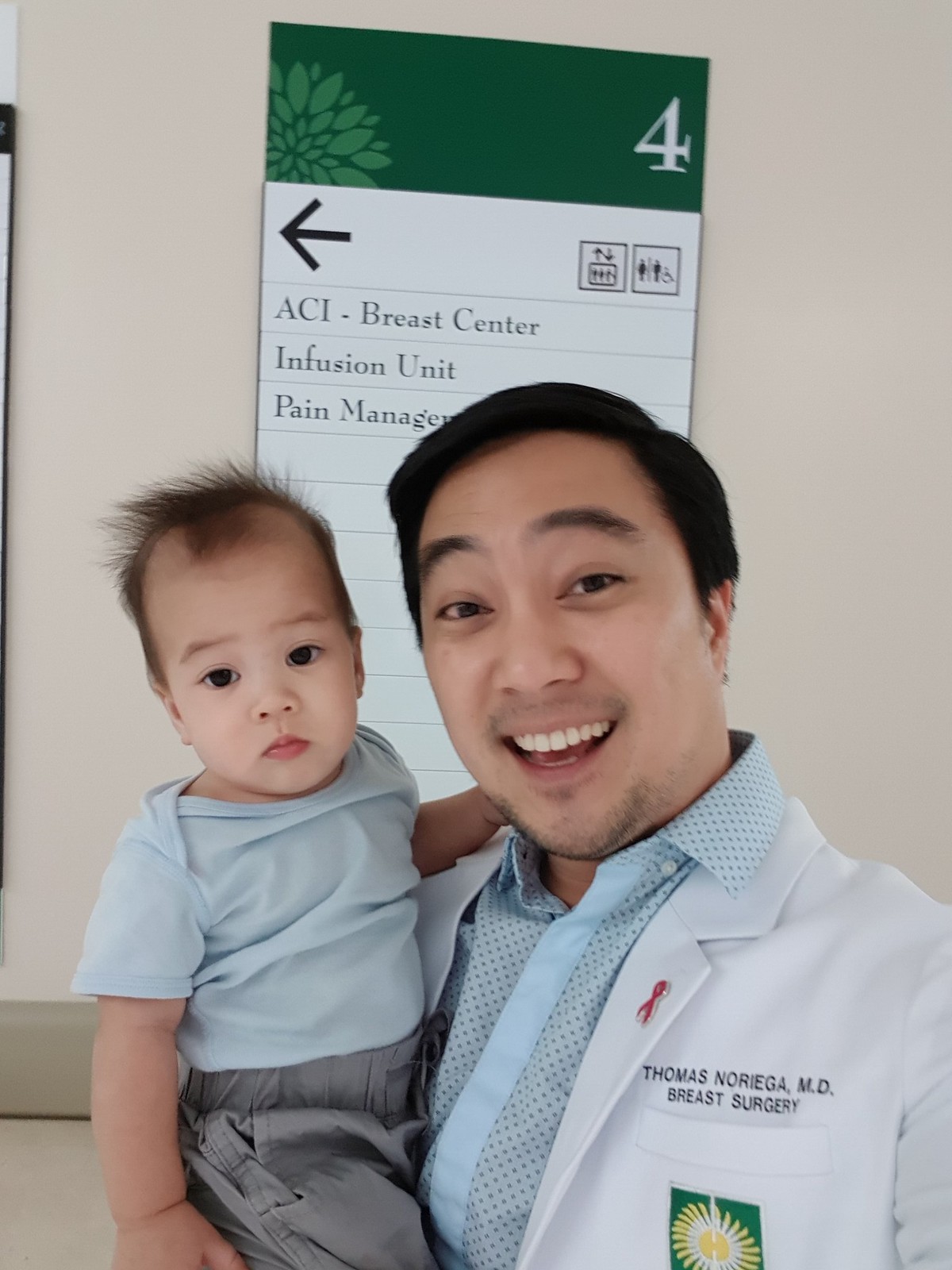In this detailed photograph taken indoors, a smiling doctor of Asian descent is captured mid-chest up, wearing a white lab coat over a light blue, polka-dotted, button-up shirt. The lapel of his coat bears a red ribbon pin, and on the chest pocket, it reads "Thomas Noriega, MD, Breast Surgery." Dr. Noriega, with short black hair, raised black eyebrows, and a five o'clock shadow, is holding a young Asian toddler. The toddler, dressed in a light blue onesie and gray pants with wispy black hair, stares blankly at the camera from the doctor's right arm. The wall behind them is light brown and adorned with a rectangular directional sign. This sign has a green background with a large white number "4" at the top, followed by a black arrow pointing to the left and the text "ACI Breast Center, Infusion Union, and Pain Management" listed underneath. The perspective suggests that the photo might be a selfie taken by Dr. Noriega himself.